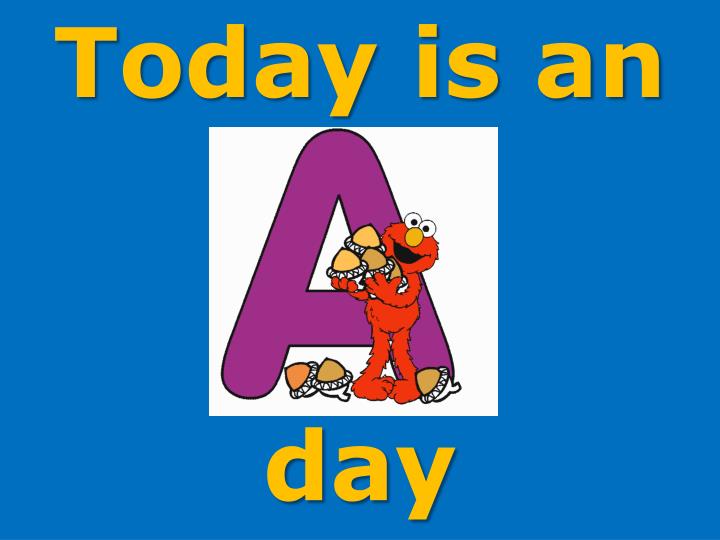The image features a solid blue background, reminiscent of a clear sky. At the top in large, bold yellow text, it reads "Today is Ann." Below this text is a centered white square. Inside the white square, the Sesame Street character Elmo, with his bright red fur, orange nose, and white eyes with black pupils, is depicted standing on the ground. Elmo's mouth forms a cheerful smile, and he is holding a bunch of acorns, four or five in total, in his hands. Behind Elmo is a large, stylized letter 'A' in rich violet or magenta color. Scattered around him on the floor are three more acorns — two to his left and one to his right. At the very bottom of the image, in the same yellow font as the text at the top, it reads "day," completing the phrase across the image as "Today is an A day."